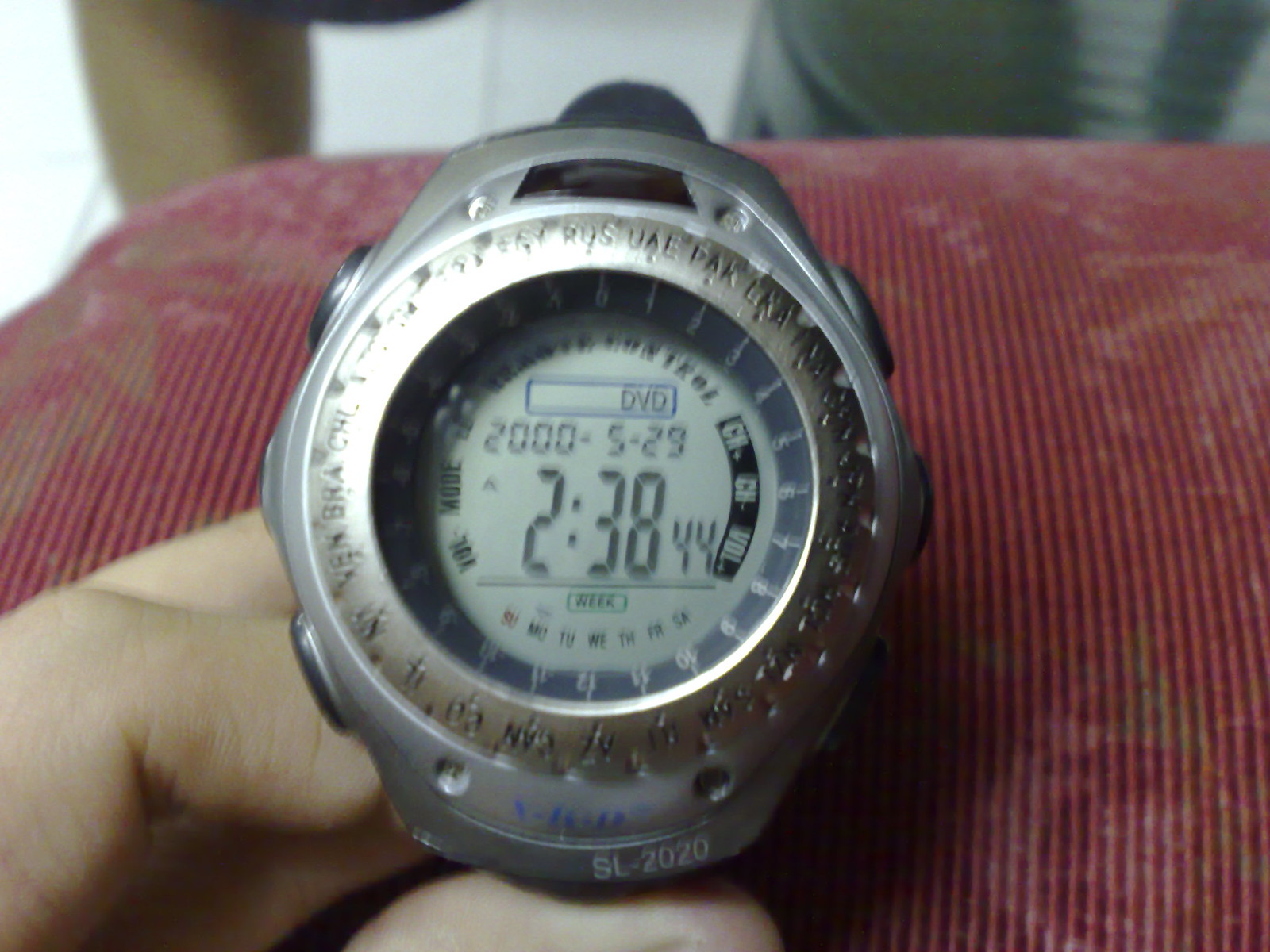A detailed photograph captures a hand with light-colored skin holding a silver, slightly bulky digital watch in the center of the frame. The watch, which is the main focus, features an engraved bezel with letters like S-U-A-E, P-A-K, and L-N-A. Some parts of these engravings are hard to read due to the darkened area on the right side and an overly bright spot on the top left. The digital display shows the numbers "2,529" and the time "2:38 PM" with 44 seconds. At the bottom of the watch face, the day of the week is displayed, accompanied by additional small numbers around the edges. This hand and watch rest on a red cloth surface, which adds a rich, textured backdrop. The background beyond the cloth surface is slightly blurred, offering a glimpse of the room without distracting from the central subject.